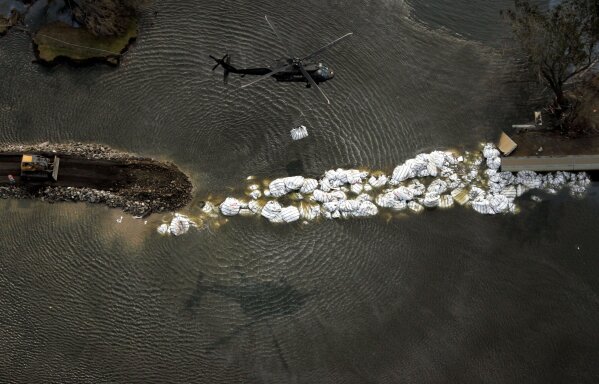The color photograph, taken from a drone in landscape orientation, captures an aerial view of a levee in New Orleans, which was breached by Hurricane Katrina 18 years ago. The levee shows signs of a partial blockage with large white masses that resemble styrofoam or concrete blocks. A Blackhawk helicopter is prominently featured at the top of the image, flying towards the right while carrying a piece of cargo—likely another one of the white objects mentioned—underneath it, presumably to be dropped as part of ongoing flood control efforts. The helicopter's reflection shimmers in the water below, adding a dynamic element to the scene. 

To the left, midway down the image, a bulldozer appears to be aiding in the construction or reinforcement of the levee. There are also a few land masses to the right and the top left, with a concrete jetty visible on the right side opposite the bulldozer. The overall style of the image is photographic representationalism, emphasizing realism and the utilitarian aspects of drone photography to document critical infrastructure repair and flood mitigation activities.